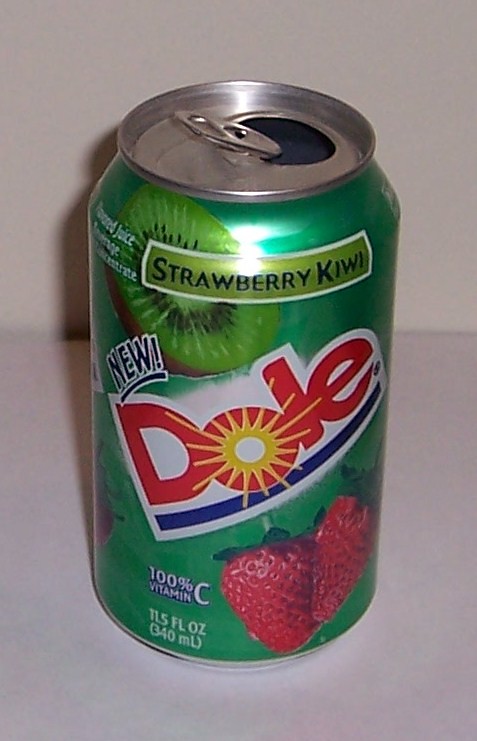This photograph features an 11.5-ounce Dole can of strawberry kiwi juice placed on a white table against a white wall. The aluminum can is open, and its design prominently showcases various elements. The can's label is green, with "Strawberry Kiwi" written in black font at the top center. Directly underneath the flavor text is an illustration of a partially cut kiwi. Below the kiwi, the word "new" is emblazoned in blue letters with an exclamation point. The brand name "Dole" is positioned mid-can, printed in red font with a distinctive yellow sunburst emanating from the "O." Beneath this, a navy blue line separates the branding from a graphic of two strawberries at the bottom of the label. To the left of the strawberries, the text "100% Vitamin C" is noted, and just below this, the volume is stated as "11.5 fluid ounces" (or 340ml). The can casts a shadow, adding depth to the otherwise minimalist setting.